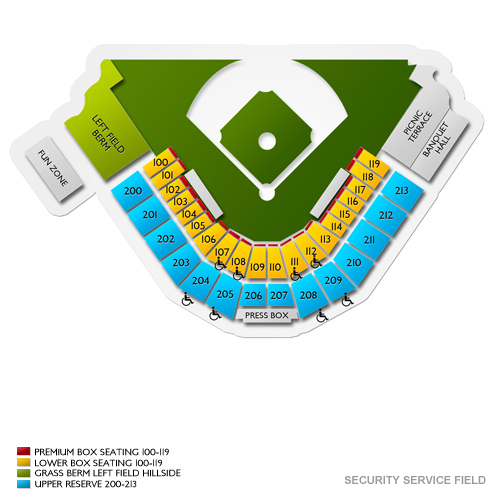This image depicts a simplified map of a baseball stadium. The map illustrates the layout of the stadium, bleachers, and signage indicating various sections. The bleachers in the first row, labeled 100-119, are color-coded in yellow and have designated handicapped spots at sections 117, 108, 111, and 112, located approximately in the middle of the row. Above and below this first row are sections labeled 200-213, where each box in these sections is twice the width of the boxes in the 100 section and colored blue. Centrally positioned in the blue section is the press box.

At the lower part of the map, the areas labeled "Security" and "Service Field" are visible. The map includes a color key for different seating areas: red indicates premium box seating found on the sides of the 100 sections, yellow denotes lower box seating, green signifies the grass berm in the left field hillside, and another shade of yellow represents upper reserved seating.